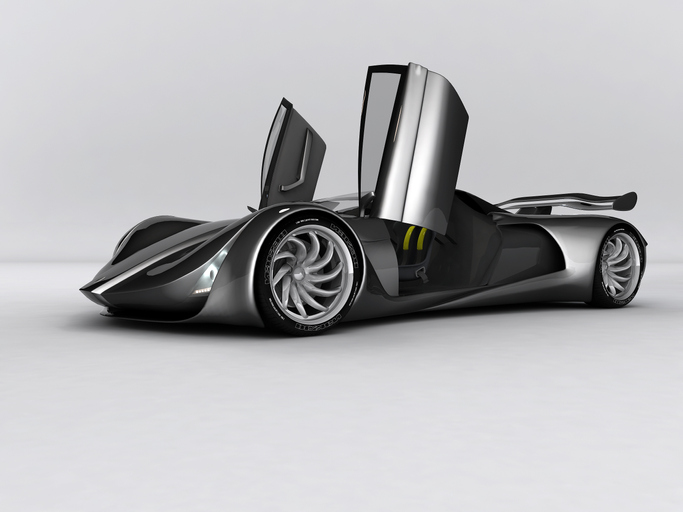This photograph captures a sleek, futuristic silver sports car against a stark, off-white background. The car features distinctive butterfly doors that tilt and rotate upwards vertically, both of which are shown in the image. Its aerodynamic design and smooth curves evoke a concept car or a vehicle straight out of science fiction, reminiscent of the iconic Mach 5 from Speed Racer. The car sits low to the ground, enhancing its sporty and exotic appeal. It boasts large, spirally steel rims and a prominent silver spoiler at the rear, reinforcing its race car-like appearance. The black interior is partly visible, including the driver's seat. There is some indiscernible text on the wheels, adding to its detailed, high-tech aesthetic.